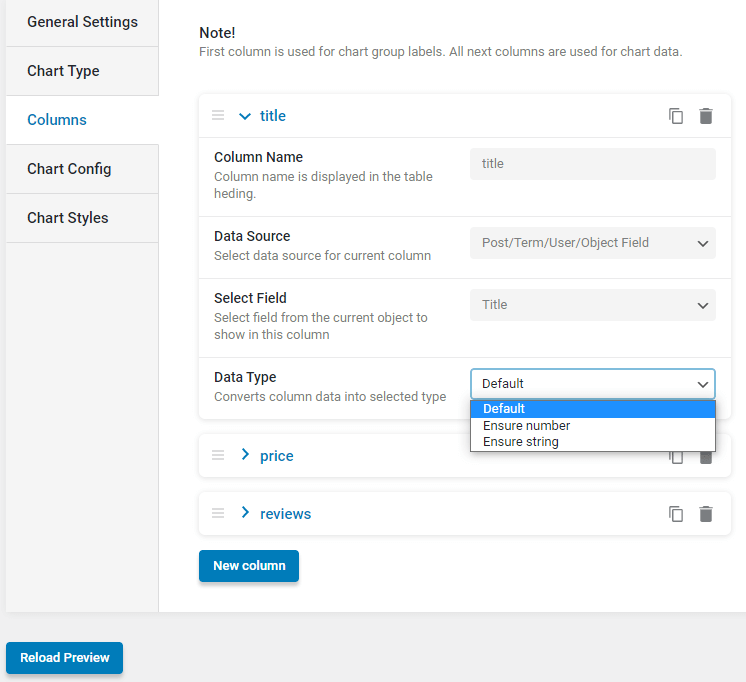The image showcases a software interface featuring a dual-pane layout. On the left side, there is a settings pane with various configuration options such as "General Settings," "Chart Type," "Columns," "Chart Configuration," and "Chart Styles." The interface is currently focused on the "Columns" section. Instructions on the right indicate that the first column is designated for chart group labels, while the subsequent columns are used for chart data.

The right pane illustrates a detailed view of the columns' arrangement, showing options to set the column name, data source, and select fields from the current object to be displayed in each column. The "Data Type" drop-down menu offers choices like "Default," "Int Number," and "String," with the default option currently selected. Additional settings are available but remain collapsed under categories labeled "Price" and "Reviews."

To finalize the setup, the user must click a blue "New Column" button. Although the specific software is not identified, the interface appears to be designed for creating and configuring detailed charts.